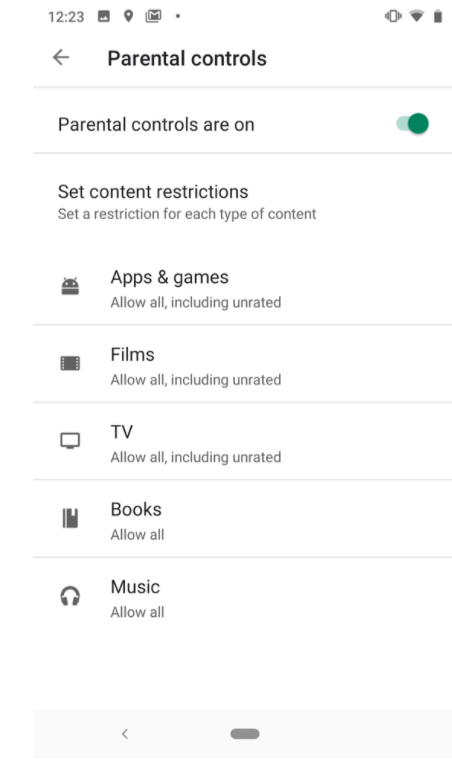This screenshot captures a parental controls settings page from a mobile device, either a phone or a tablet. At the very top, the device status icons are displayed, showing it is 12:23 p.m. The status bar also indicates the presence of mail notifications, active vibration mode, Wi-Fi strength at approximately 75%, and a nearly full battery.

Directly below the status bar, the title "Parental Controls" is prominently displayed, accompanied by a back arrow, suggesting users can navigate to the previous screen by tapping the arrow.

The main content of the page starts with a toggle switch labeled "Parental Controls are on," which is set to the "on" position, as indicated by its green color.

Further down, a section titled "Set Content Restrictions" allows users to define access levels for various content types. This section includes the following categories:

1. **Apps and Games**: Allow all, including unrated content.
2. **Films**: Allow all, including unrated content.
3. **TV**: Allow all, including unrated content.
4. **Books**: Allow all content.
5. **Music**: Allow all content.

At the bottom of the screen, there's a gray horizontal scroll bar, indicating that the page can be scrolled from left to right, although no additional visual elements are present beyond the described content. This provides a simple yet comprehensive overview of the parental control options available on the device.